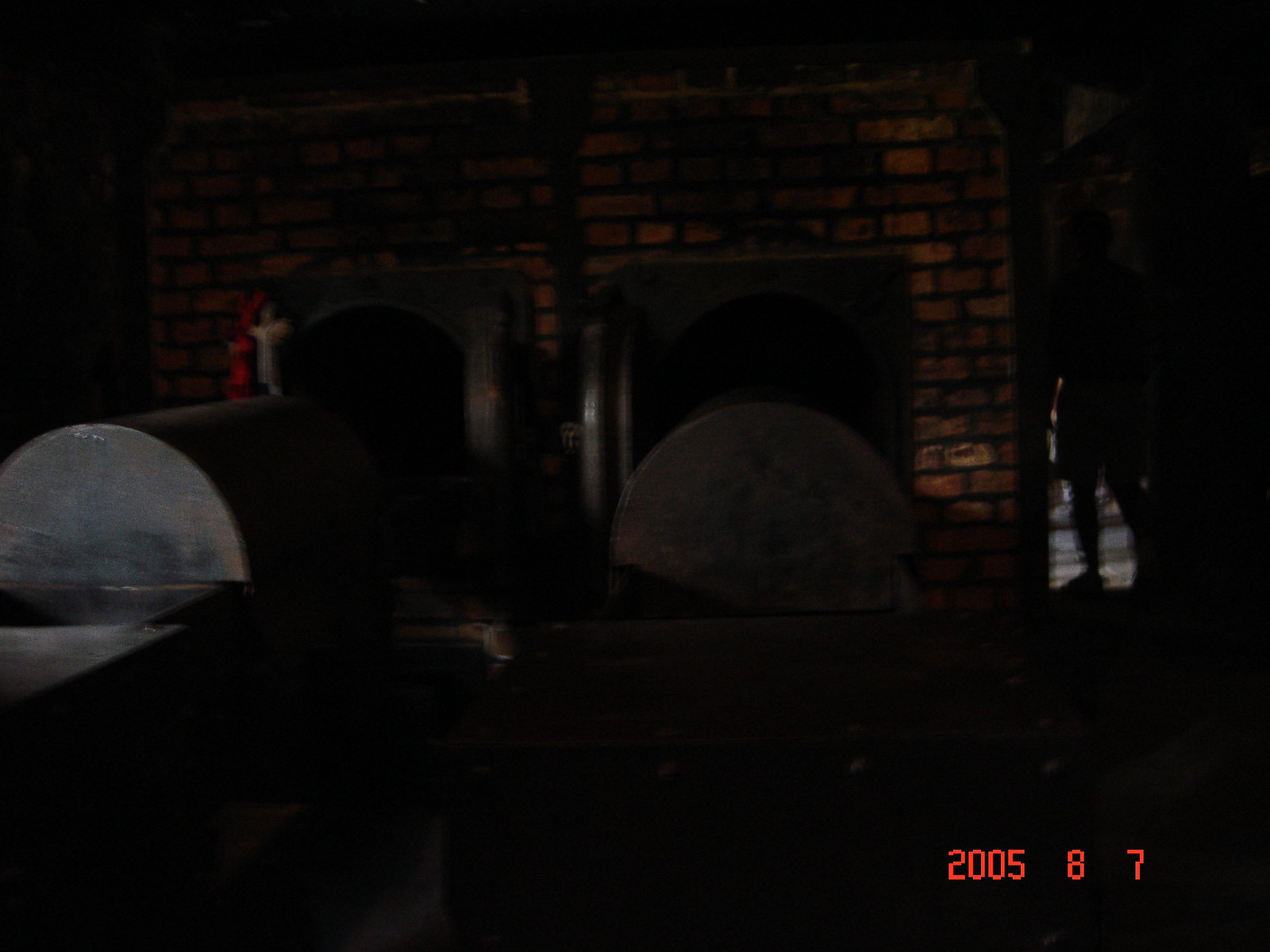The image, timestamped "2005 8 7" in red digits at the bottom right corner, appears to capture a somber scene in a dimly lit crematorium. The main focus is on two red and brown brick furnaces, each featuring square outlines with circular centers designed to house round-shaped black metal tubes that slide out in front. These tubes, segmented with a handle on the back and able to open up via a center cut, are part of the metal furnace apparatus which also has closable doors. The furnaces’ blackened interiors are stark against the bricks, indicating where fires would typically burn. Amidst the shadowed surroundings, a silhouette of a man standing in a doorway to the right adds to the eerie atmosphere. The image is dark overall, with hints of reflections and obscured shapes, suggesting possible digital capture and challenging visibility.